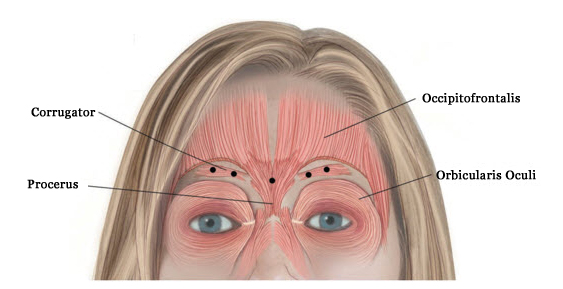This image is a detailed textbook diagram of the upper part of a middle-aged woman's face, showcasing the muscles and anatomical features from the tip of the nose up. The woman has blonde hair with brown highlights, and blue eyes. The diagram highlights specific facial muscles with different colored tones, including two shades of pink around the forehead and eyes. Key muscles are labeled with black lines pointing to various areas: the occipital frontalis on her right forehead, the corrugator around the eyebrows, the orbicularis oculi near the right eye, and the procerus at the bridge of the nose. This educational illustration provides a clear view of the facial structure, emphasizing the underlying musculature.